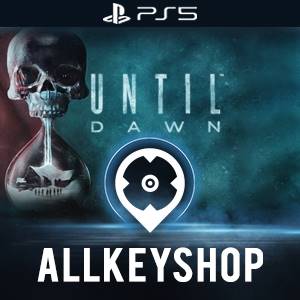This digital image represents the cover art for a PS5 game titled "Until Dawn." At the top, a black banner features the PlayStation logo accompanied by the text "PS5." Dominating the left side of the cover is an intricate design, where the top element is a skull, seamlessly transitioning into an hourglass shape beneath it. Inside the hourglass is a snow-covered cabin roof with shadowy figures standing in front of it, evoking a chilling night setting. A prominent target-like symbol—a circle with a cross pattern—appears above the bottom section. At the very bottom of the image, another black bar displays the text "All Key Shop" in bold, white capital letters. The entire background conveys a blue, night sky ambiance, enhancing the eerie and mysterious atmosphere of the game.